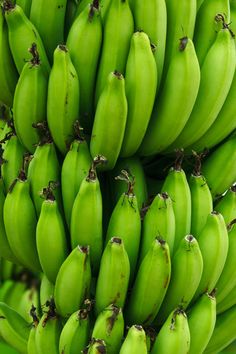The image showcases a dense, close-up view of an extensive bunch of green plantains. The plantains are all consistently green with varying shades, including a light, almost lime-green hue. Each plantain is oriented upwards, displaying black tips and stems at their top ends, creating a naturalistic and unaltered appearance. The plantains are tightly clustered together, forming rows with the smaller and shorter ones at the bottom and the longer, more mature ones at the top. The background lacks any identifiable context, offering no textual or environmental clues, merely a slightly blurry continuation of the green plantains. The overall composition highlights the freshness and unripe state of the plantains, not yet ready for consumption.